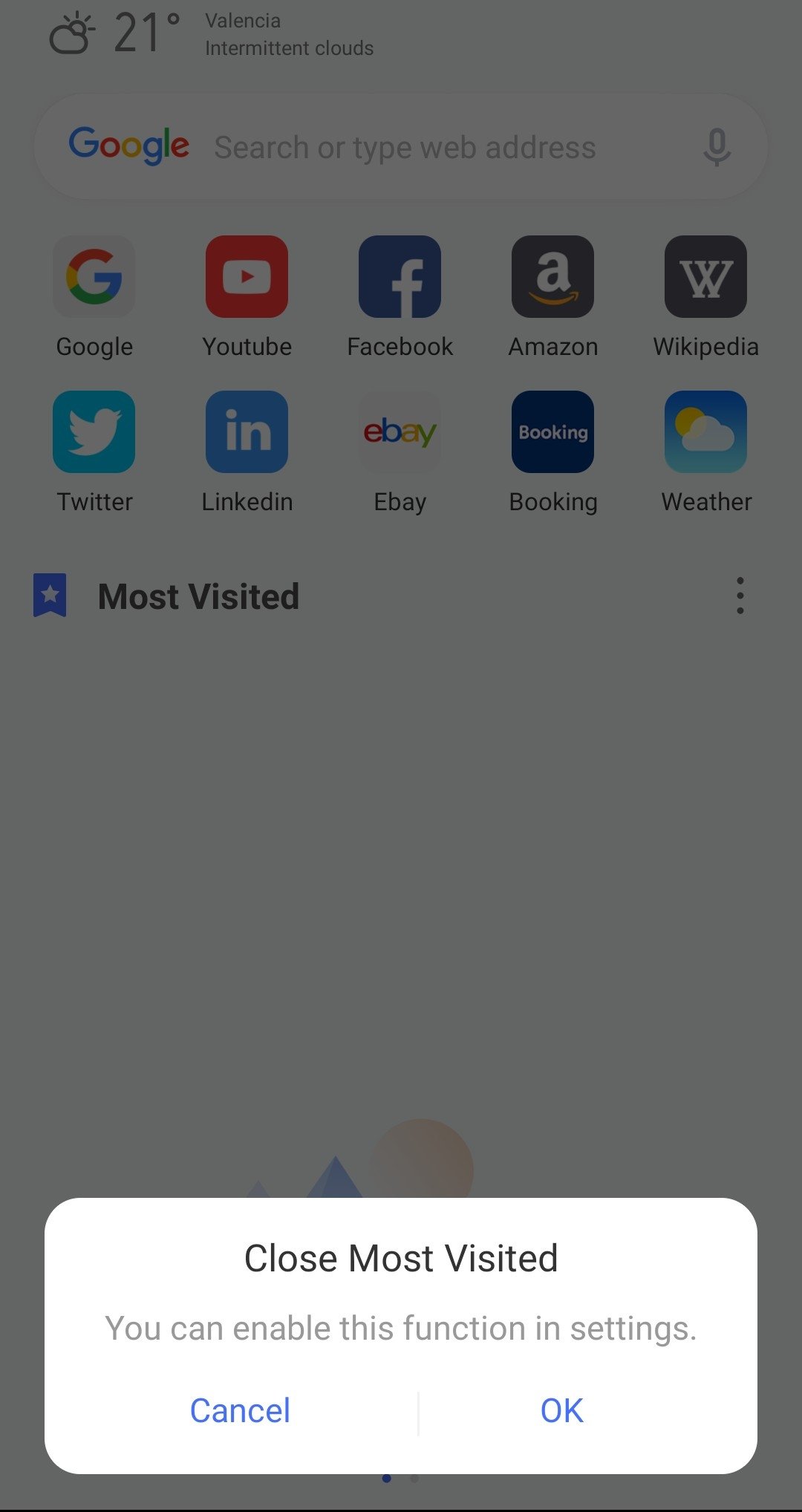The image appears to be of a smartphone screen, although it is not explicitly clear. The display shows a partly sunny weather forecast for Valencia, indicating a temperature of 21 degrees and intermittent clouds at the top. Directly beneath this is a Google search bar, featuring the iconic Google logo in blue, red, yellow, and green.

Below the search bar, there are two rows of icons representing popular apps and websites. The top row includes icons for Google, YouTube, Facebook, Amazon, and Wikipedia, while the bottom row features Twitter, LinkedIn, eBay, Booking.com, and an app related to weather. Each row contains five icons.

The entire screen is covered by a gray film that mutes the colors, giving it a subdued appearance. At the bottom of the screen, a white horizontal rectangle notification has popped up. This notification says, "Close most visited. You can enable this function in settings," with options to "Cancel" or "Okay" displayed in blue text.

The app icons predominantly feature colors such as red, blue, yellow, and green.